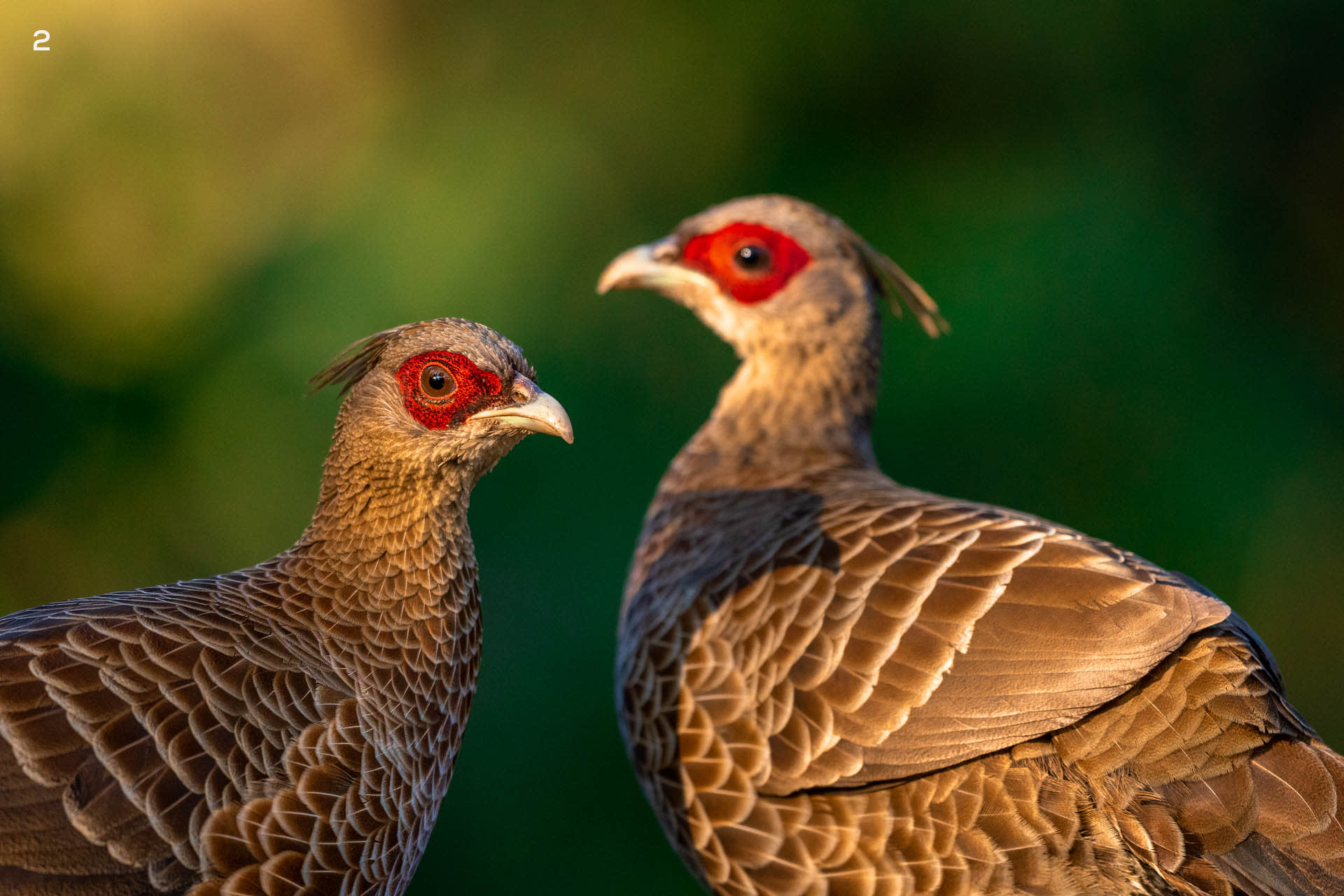In this striking photograph, two medium-sized birds stand against a blurred green and brown backdrop, likely in a forest setting. The birds, which could be quail or a related species, have predominantly light to medium brown feathers with intricate details that appear almost surreal in their clarity. Notably, their sharp, off-white beaks are slightly curved, adding to their distinctive appearance. The focal point, however, is the bright red patches encircling their brown eyes, giving them a striking, mask-like appearance. One bird faces to the right while the other faces to the left, each presenting a side profile with only one eye visible to the camera. The feathers around their tails feature a mix of brown and golden hues with darker accents, and a small tuft of feathers on their heads extends slightly to the back. The more focused bird on the left even casts a shadow upon the slightly larger one on the right, adding depth to the image. The overall contrast between the vivid green background and the rich, detailed markings of the birds makes for a captivating and beautiful scene. The image also contains the number "2" in the top left corner, with no other text present.